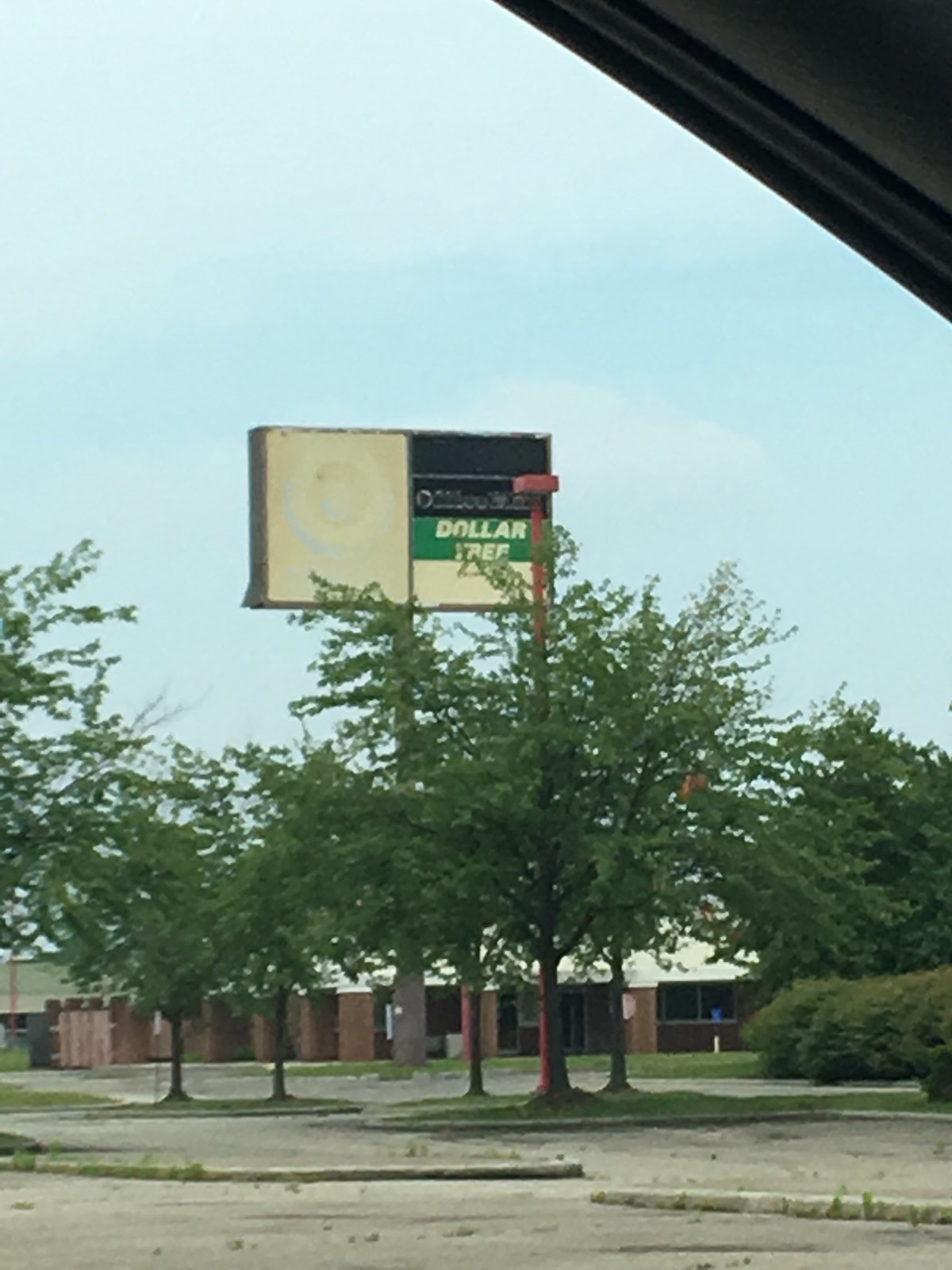An empty parking lot of what appears to be a defunct strip mall or small shopping center dominates the scene. At the forefront stands a tall marketing sign mounted on a large cylindrical post. The sign is divided into several sectioned areas. The left half is a blank white space. The right half features a striped design in black, green, and white, with the only visible text being "Dollar Tree" in white letters against the green section. The rest of the sign remains blank.

Surrounding the parking lot are islands of grass, bordered with distinct curb lines. The grass appears well-trimmed and meticulously maintained. In the background looms a short brick building, characterized by brick pillars that support a light-colored overhang, providing shade to the storefronts below. The parking lot itself is devoid of vehicles, with scattered debris, likely from grass clippings, visible on the asphalt. The overall scene conveys a sense of abandonment and stillness.